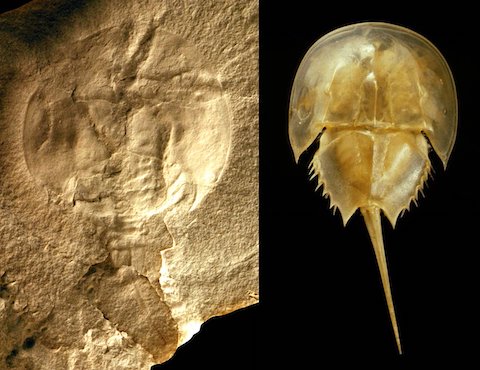The image displays a detailed comparison between a modern horseshoe crab and its ancient fossil counterpart. On the right side, set against a stark black background, lies a living or contemporary horseshoe crab, exhibiting a tannish yellow color with a prominent, elongated, pointed tail. On the left side, almost symmetrically split down the center of the image, is the fossilized impression of a horseshoe crab embedded in a tan-brown rock foundation, vividly preserving the outline of its body. The fossil captures the creature's distinctive shape and features, reminiscent of an era when such animals thrived. The juxtaposition in the image highlights both the preserved artifact's geological context and the living organism's anatomy, emphasizing the fossil's importance in reconstructing the historical appearance of this ancient species.